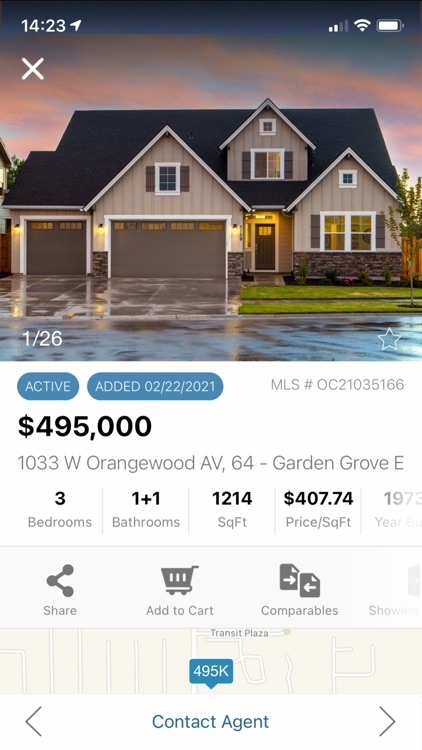This screenshot, taken at 2:23 p.m. on a mobile device connected to Wi-Fi with almost full battery, captures an app listing for real estate properties. Dominating the screen is a large image of a two-story suburban home, typical of an American city. The house features a dark black roof, tan or beige paneling, and a brick façade covering the lower half of the first floor. The photo appears to have been taken during or just after a storm, as evidenced by the wet driveway and street that reflect ambient light. The outdoor lights of the house are illuminated.

The house is listed for sale at $495,000 and is located at 1033 West Orangewood Ave, Unit 64, in Garden Grove. The property details indicate that it comprises three bedrooms and 1.5 bathrooms spread across 1,214 square feet, translating to a price of approximately $407.74 per square foot.